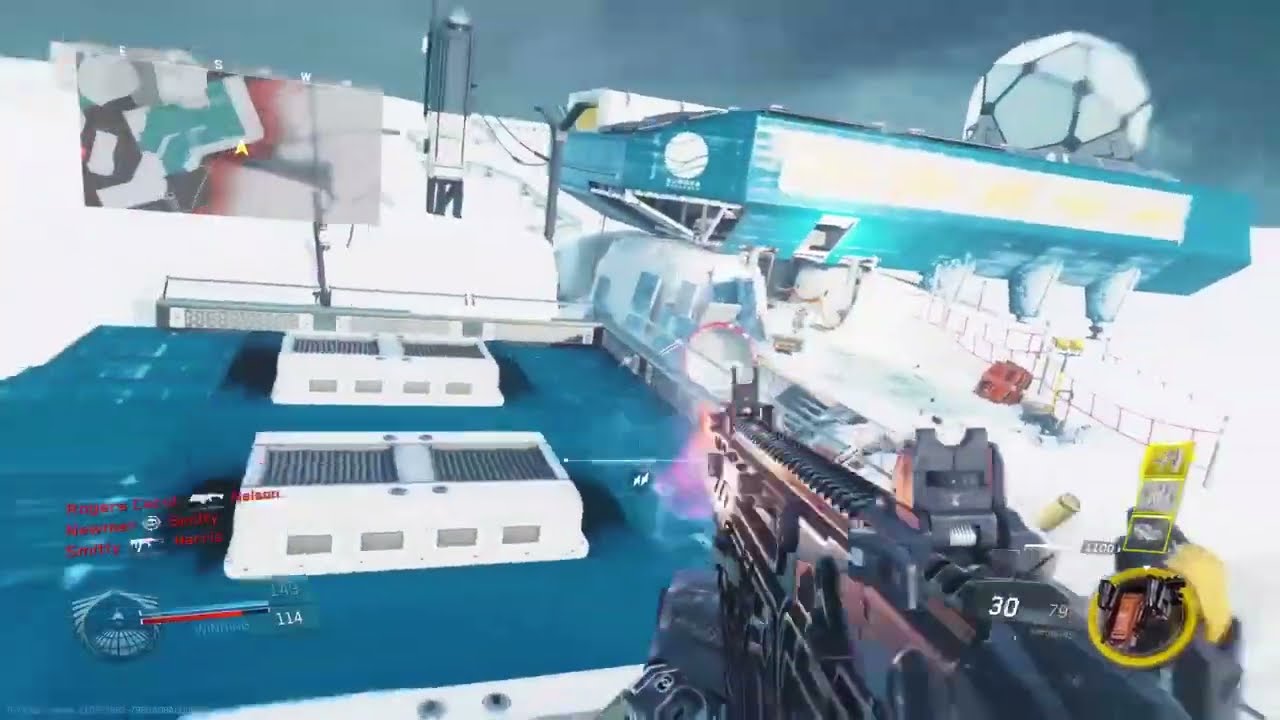The image is a screenshot from a first-person shooter video game. The player is holding a large black machine gun with a slight tint of red, which extends out from the bottom right corner. The player's left hand, glowing black, grips the front of the gun. In the immediate firing zone and towards the right-hand side, a yellow circle with protruding gears is visible, possibly a targeting or HUD element. The environment appears to be a marine vessel with a blue floor. Centered in the image are two white rectangles, each topped with gray grates. These structures resemble vents and are slightly raised from the floor. In the background, at the top right corner, a large white sphere akin to Disney World's Epcot Center stands out, outlined in black. The far end of the platform is bordered by a white wall, and there are also various antennas and possibly other structures or towers in the scene. Additionally, a score card and game-related text and codes appear within the frame.